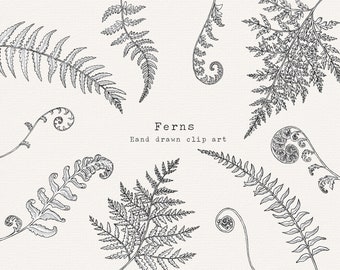The image is an intricately detailed, pencil-drawn artwork showcasing around 10 different types of ferns arranged symmetrically around a white background. The ferns, appearing in a dark graphite grayscale, frame the edges of the picture with their tips pointing inward toward the center. In the very center, "ferns" is prominently typed, alongside the words "drawn clip art." The composition includes four unique ferns at the top, two ferns on each side, and four more ferns at the bottom. Some of the ferns feature long stems with pairs of leaves on each side, while others have more leaves or exhibit a curly structure. The detailed side-view illustrations showcase the intricate details of each fern, emphasizing their unique characteristics while maintaining a cohesive, botanical theme.